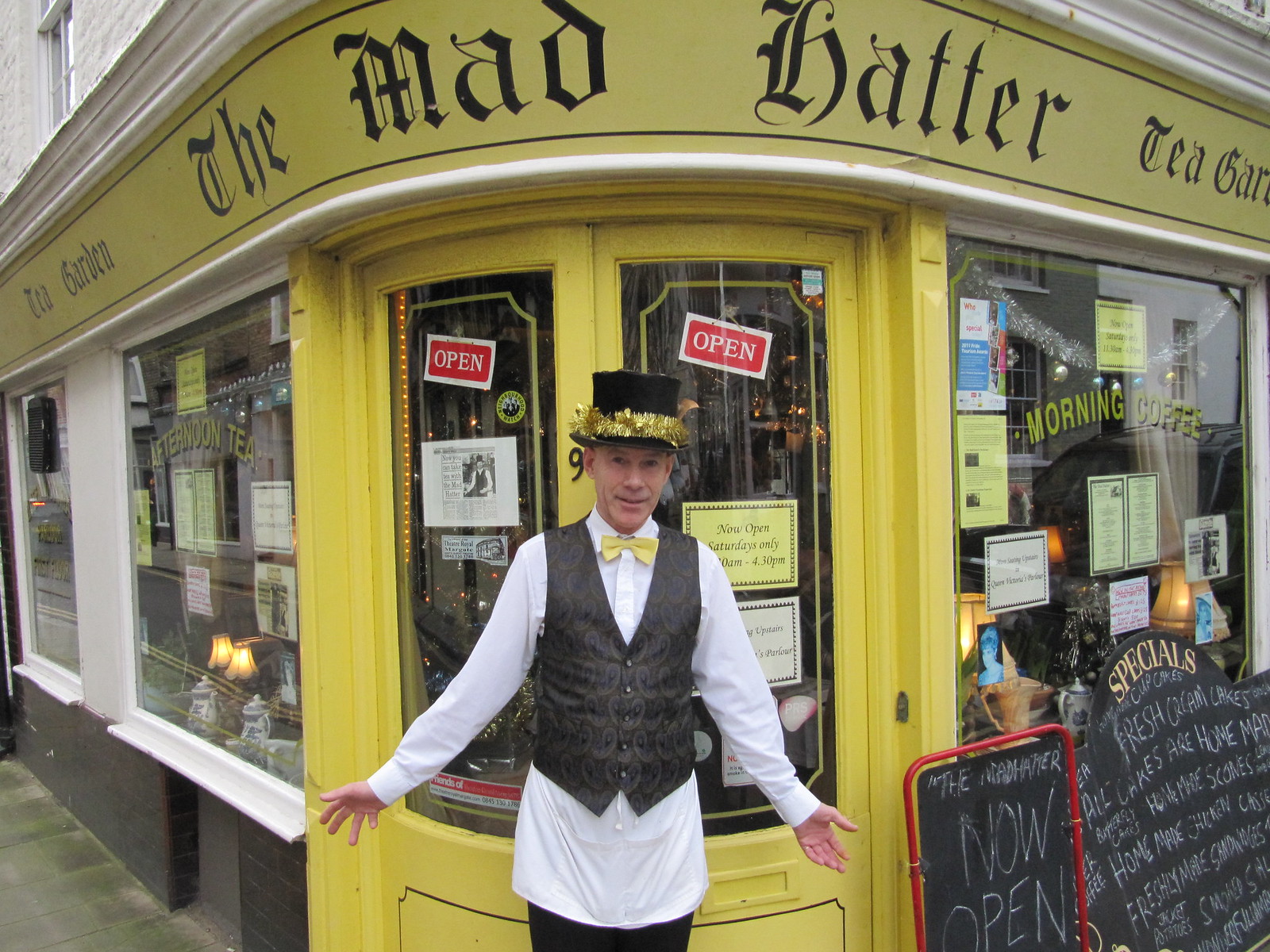In this vivid image, we see a man joyfully standing with his arms outstretched in front of a place called "The Mad Hatter." This establishment appears to be a charming tea shop situated in a business district. The building’s exterior is painted bright yellow, with the name "The Mad Hatter" prominently displayed in gothic, old English black font. The front doors are adorned with red "Open" signs, signaling that the place is welcoming customers. To the side, chalkboard signs announce the shop is "Now Open" and list specials, hinting at homemade food and beverages served inside.

The man at the entrance adds a whimsical touch to the scene. He is dressed in a distinctive outfit: a black top hat embellished with a shiny golden fuzzy band, a white long-sleeved collared shirt, a gray vest with a playful repeating pattern, a yellow bow tie, and black pants. His cheerful demeanor, with a partially smiling face, matches his festive attire, which echoes the spirited nature of the tea shop. To the right window of the shop, there's an inscription "Morning Coffee," and to the left, "Afternoon Tea," enhancing the cozy and specialized ambiance of the place. The windows are bordered in white, framed by black brick below, and set against the yellow wall, contributing to the overall inviting aesthetic of the tea shop.